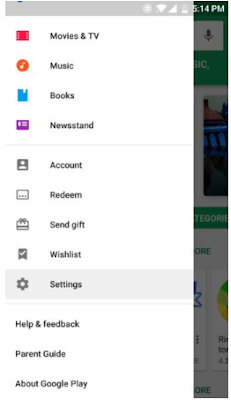Screenshot of a smartphone screen at 5:14 PM with full WiFi signal but almost dead battery. The background features a green and white pattern with grayed-out images, giving it a gray tint. A pop-up menu with a gray border on top appears on the left side, partially overlaying the screen. The menu lists various options with icons and text. The first option is a red box labeled "Movies & TV," followed by an orange circle with a music note labeled "Music." Next are a blue icon labeled "Books" and a purple icon labeled "Newsstand." Beneath these, the menu options include "Account," "Redeem," "Send Gift," "Wish List," "Settings," "Help & Feedback," "Parents Guide," and "About Google Play." One of the settings options is highlighted in light gray.